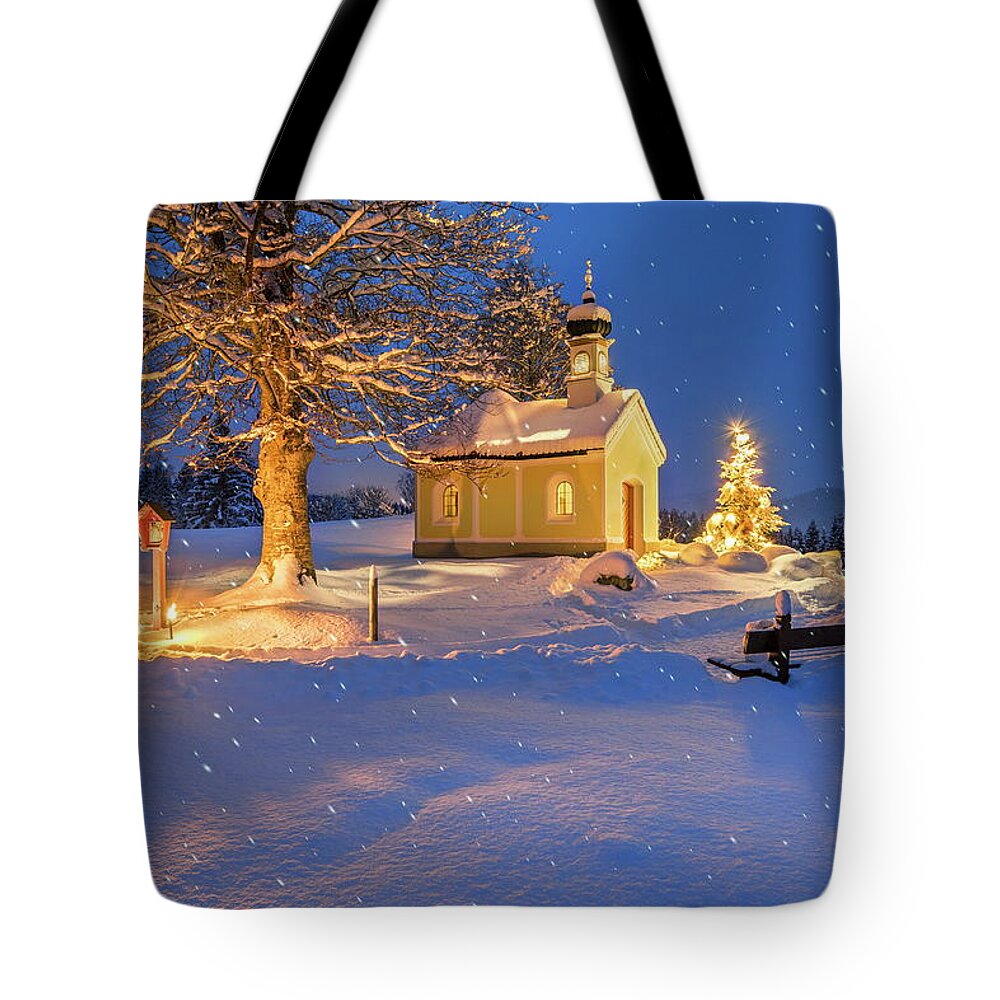This image showcases a rectangular tote bag with curved edges against a completely white background. The bag features a wintry night scene transposed onto it, covering the entirety of the surface. The tote bag itself has a black handle, partially visible at the top. Central to the image is an old white country church with a striking red door, viewed from the side, revealing its steeple topped with black and a snow-covered roof. The warm glow from the church's windows adds a cozy contrast to the snowy setting. To the right of the church stands a small Christmas tree adorned with twinkling white lights, creating a radiant effect on the bag. The foreground features a large leafless tree to the left, dusted with snow and possibly icicles, while half of a bench is visible on the right side. A red birdhouse with a black roof also decorates the left side. Snowflakes continue to fall, blanketing the ground and covering the snow-tipped trees in the background. The serene sky, lit with stars, completes this enchanting winter night scene.